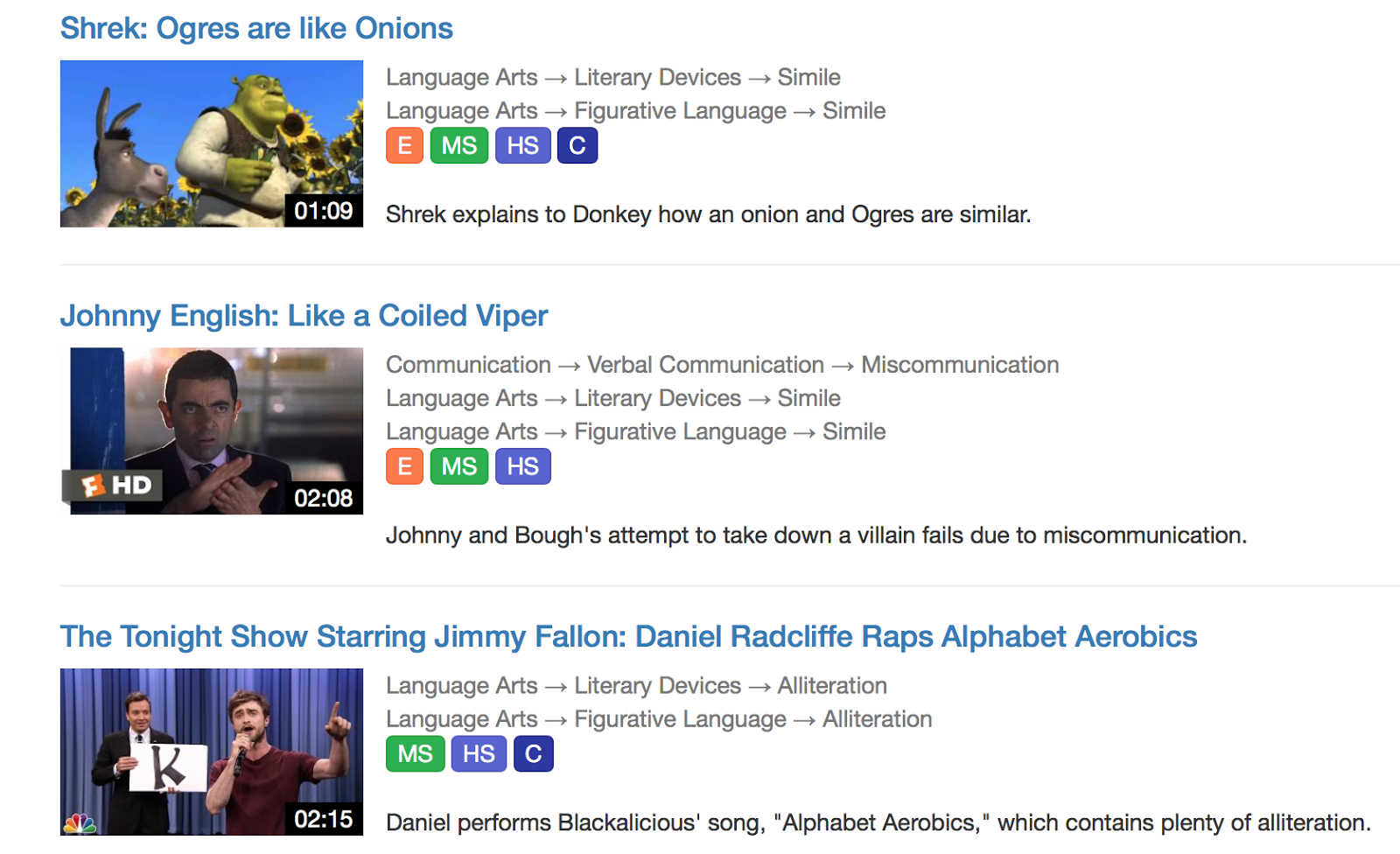**Image Description:**

The image is a screenshot from an unspecified webpage displaying three distinct listings, each with a title, image, and description. 

1. **Listing One:**
   - **Title:** "Shrek: Ogres Are Like Onions" (in blue font)
   - **Image:** A small screenshot from the Shrek movie featuring the characters Shrek and Donkey standing in a field with sunflowers in the background.
   - **Description:** This section categorizes the content under "Language Arts" and specifically focuses on literary devices, emphasizing the use of similes. 
   - **Educational Tags:** 
     - Light Red Box with Letter E
     - Green Box with "MS"
     - Purple Box with "HS"
     - Blue Box with Letter C
   - **Caption:** "Shrek explains to Donkey how onions and ogres are similar, illustrating the use of simile."

2. **Listing Two:**
   - **Title:** "Johnny English: Like a Coiled Viper" (in blue font)
   - **Image:** A headshot of a man appearing to be in his late 30s or early 40s, wearing a dark suit, white shirt, and tie. 
   - **Description:** This section touches on aspects of "Communication," particularly verbal communication and miscommunication.
   - **Educational Tags:**
     - Red Box with Letter E
     - Green Box with "MS"
     - Purple Box with "HS"
   - **Caption:** "Johnny and his team attempt to take down a villain, but their efforts are thwarted due to miscommunication."

3. **Listing Three:**
   - **Title:** "The Tonight Show Starring Jimmy Fallon: Daniel Radcliffe Raps 'Alphabet Aerobics'" (in blue font)
   - **Image:** A screenshot from an episode of The Tonight Show featuring Jimmy Fallon on the left and Daniel Radcliffe on the right. Radcliffe is wearing a maroon t-shirt, holding a microphone near his mouth, and gesturing with his other hand.
   - **Description:** This section highlights "Language Arts" focusing on literary devices, particularly alliteration.
   - **Educational Tags:**
     - Green Box with "MS"
     - Purple Box with "HS"
     - Blue Box with Letter C
   - **Caption:** "Daniel Radcliffe performs the song 'Alphabet Aerobics' by Blackalicious, which features extensive use of alliteration."